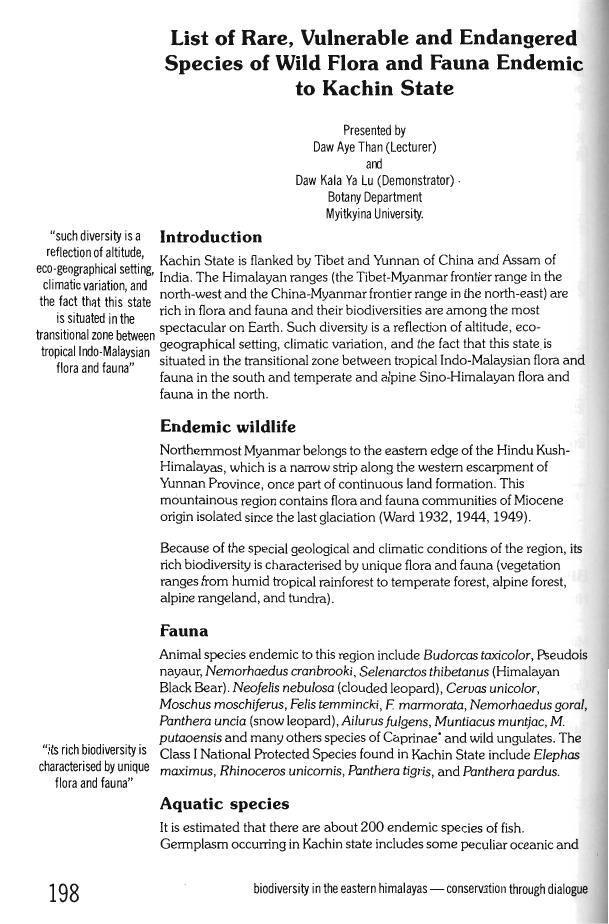This image depicts a page from a book, featuring a white background with text in black. The page is numbered 198 at the bottom left and is titled "List of Rare, Vulnerable, and Endangered Species of Wild Flora and Fauna Endemic to Kachin State" at the top in bold. The introduction highlights the geographical and ecological diversity of Kachin State, which is bordered by Tibet, Yunnan of China, and parts of India. The region, encompassing the Himalayan Ranges, the Tibet-Myanmar Frontier Range in the northwest, and the China-Myanmar Frontier Range in the northeast, boasts a spectacular biodiversity due to its varied altitude, unique ecogeographical setting, and climatic variation. The text is presented by Da A, then a lecturer, and Da Kala Yalu, a demonstrator from the Botany Department of Metikinyina University. The introduction emphasizes how the state's location in a transitional zone between tropical Indo-Malaysian flora and the temperate, alpine Sino-Himalayan fauna contributes to its rich biodiversity. Below the title, there's a series of paragraphs, including one on endemic wildlife, fauna, and aquatic species, each detailing different aspects of the region's biodiversity.